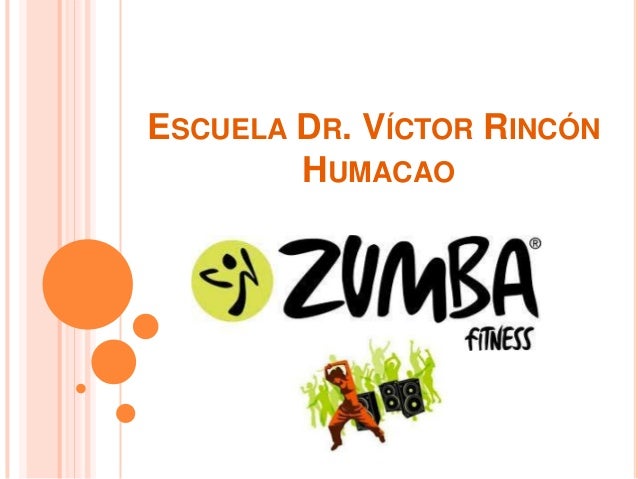This is a business card set against a pristine white background, prominently featuring a vertical light pink border with orange circles running from top to bottom along the left edge. These circles decrease gradually in size as they descend. At the top center, in bold orange capital letters, it reads "ESCUELA DR. VICTOR RINCON HUMACAO." Beneath this text lies a green olive circle adorned with a black Zumba logo. Alongside the logo, "Zumba" is inscribed in black, and below it, the word "Fitness" appears. At the bottom, an illustration showcases a dynamic scene of green silhouettes dancing, with an orange silhouette of a woman leading the group, further enhancing the energetic vibe.